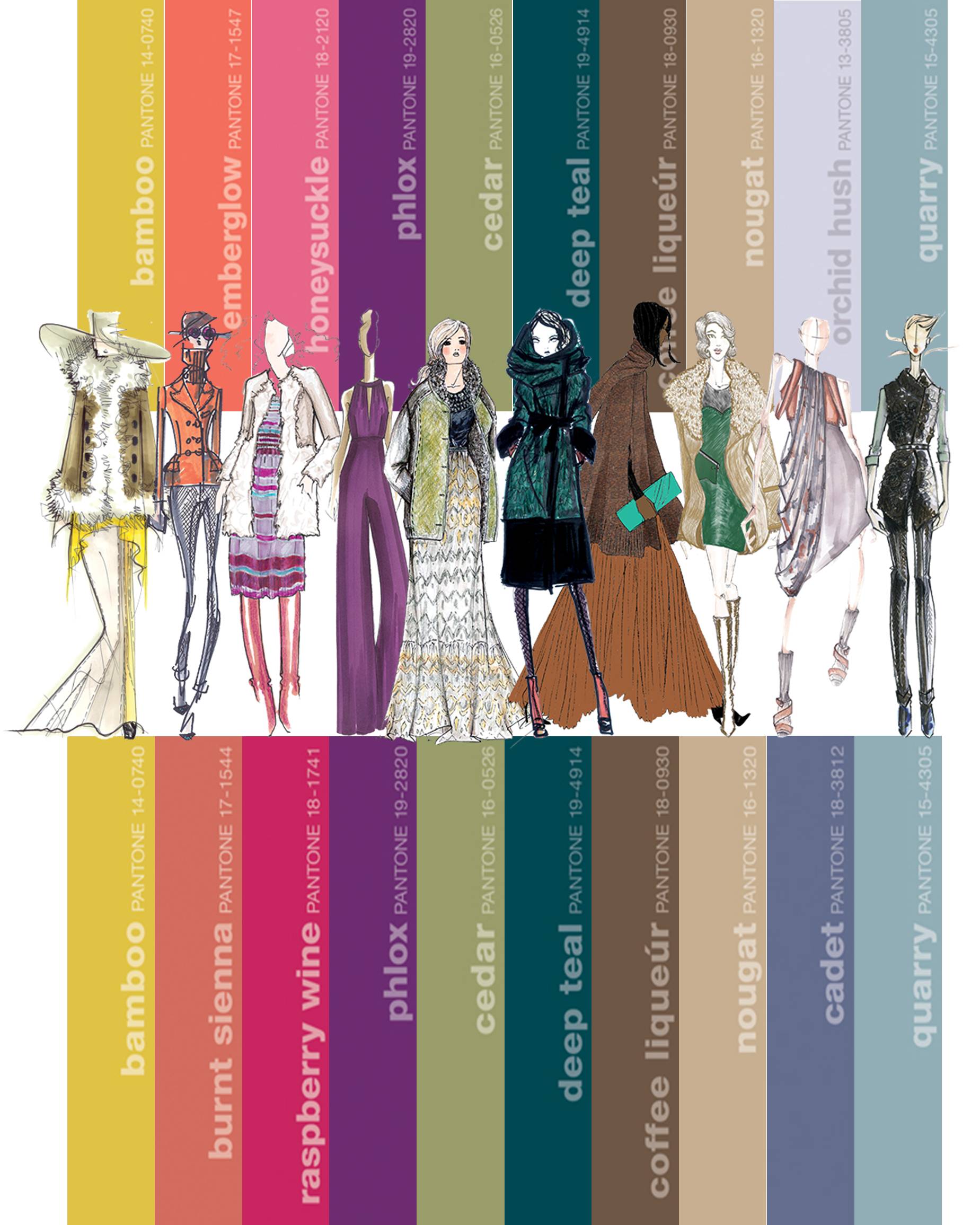This image is a detailed, rectangular illustration resembling a color palette for a fashion designer or stylist, showcasing a series of ten artificial, cartoon-like fashion sketches of women, each dressed in different colored outfits. The illustration is organized into vertical columns both at the top and bottom, each representing a unique color. Starting from the left, the first column features a woman in a yellow, fur-lined jacket and long skirt labeled "Bamboo." Next is a woman wearing an "Ember Glow" colored jacket, followed by a woman in a "Honeysuckle" dress paired with "Raspberry Wine." The fourth column presents a woman in a sleeveless, dark purple jumpsuit labeled "Phlox." 

Next, a woman dons a "Cedar" colored vest over a dress, while another wears a "Deep Teal" coat over her dress. Then, a woman is seen in a "Coffee Liqueur" brown outfit, followed by one in a beige "Nougat" jacket. The penultimate figure showcases "Orchid Hush," a light gray ensemble, and finally, the last column features "Quarry," a gray jacket with matching undersleeves. Each corresponding color is labeled with both its name and an illustrative sketch, making this a comprehensive visual representation of the various colors within a fashion-themed setting.